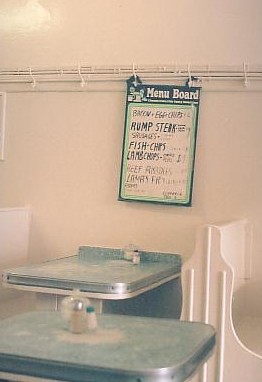The image shows an interior space adorned with a white, wooden wall that dominates the background. At the top center of the image, a white, metal shelf-like structure is affixed to the wall, featuring five hooks evenly spaced out horizontally. A poster hangs from the third and fourth hooks, suspended by its corners. The poster has a striking green background and is titled "Menu Board" in white text. A light green vertical rectangle is present on the poster, containing a list of food items written in black text: rump steak, fish & chips, and lamb chops.

In the foreground, the establishment appears to be a dining area with tables and chairs. The dining chairs are primarily white and made of plastic, with one white chair visible on the bottom right and the back of another on the bottom left. Additionally, a few chairs with greenish-teal accents can be seen in the center and bottom middle of the image. Each table is neatly set with salt and pepper shakers, emphasizing the readiness for diners.